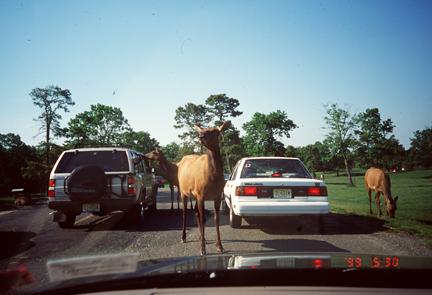In this rectangular photograph, an outdoor scene unfolds, reminiscent of a drive-through safari. Captured through a windshield, the image reveals two vehicles ahead—a vintage Volvo on the right and a silver SUV on the left—traversing a gravelly road. Surrounding these vehicles are stately, brown deer, their long legs and upright ears clearly visible. One deer stands center frame, gazing forward, though the image is slightly blurry and grainy. To the right, near the Volvo, a deer lowers its head to graze, while on the left, another deer extends its head inquisitively toward the SUV's window. The backdrop features a lush green field interspersed with trees. In the lower right corner, a timestamp reads "09 09 5:30," presumably indicating the date is September 9, 1999.